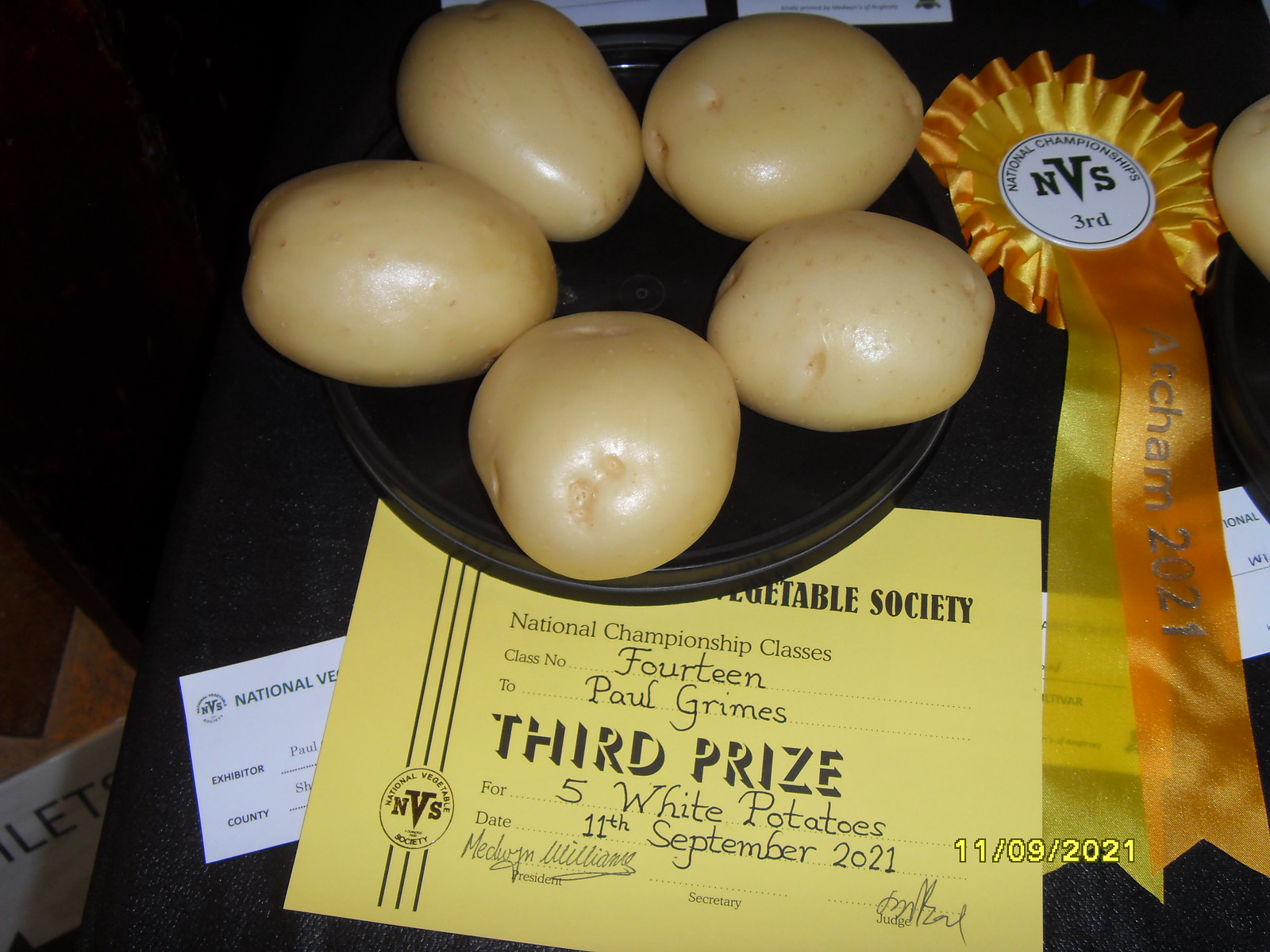The landscape-oriented color photograph showcases a plate with five round, shiny, and smooth unpeeled white potatoes, prominently positioned at the top center of the image. Accompanying these potatoes is a golden ribbon with a white circle in the middle, emblazoned with the letters "NVS" and the word "Third" underneath. Partial visibility reveals a yellow prize card beneath the plate, detailing Paul's achievement. The top of the card reads "Vegetable Society" and "National Championship Classes," with the handwritten details awarding "Third Prize" to Paul Grimes for "Five White Potatoes" on September 11th, 2021. The crisp, photographic realism captures the celebratory essence of Paul Grimes' third-place award.